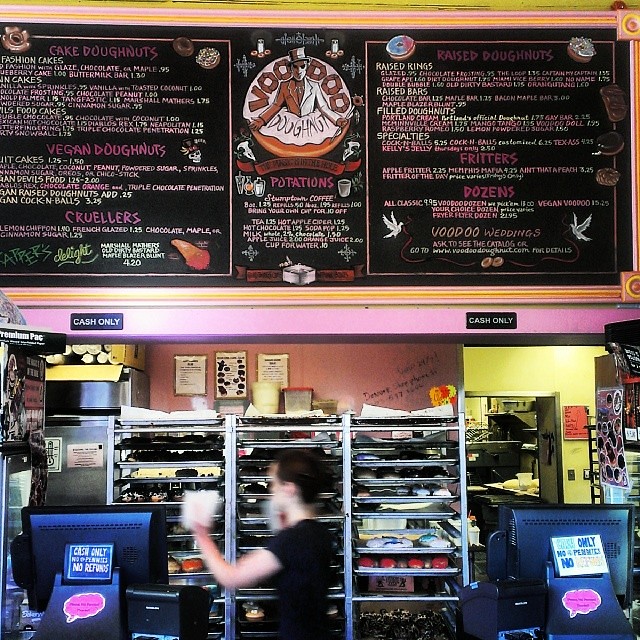The image captures a bustling scene inside a quirky bakery named Voodoo Doughnuts. Dominating the top half is a vibrant black menu board with an eclectic mix of pink, white, and green text and illustrations, set against a yellow and reddish backdrop. In the center of the board, there's an eye-catching illustration of a doughnut with a man in a white suit and top hat emerging from its center, with the words "Voodoo Doughnut" encircling the icing. The left side of the menu lists categories such as cake doughnuts and vegan doughnuts, while the right side enumerates raised doughnuts, fritters, and dozens, alongside a note about "Voodoo Weddings."

Below the menu, two black cash registers with pink and blue accents sit on the counter, one in the bottom left and the other in the bottom right. Both feature signs indicating "cash only" and possibly "no refunds." Between the registers stands a blurred figure of a person, arm raised, suggesting motion. Behind this person, metallic baking trays filled with an assortment of doughnuts are visible. To the right, an open door reveals a glimpse into a kitchen, adding depth to the image. The setting is colorful and energetic, capturing the distinctive, whimsical atmosphere of Voodoo Doughnuts.